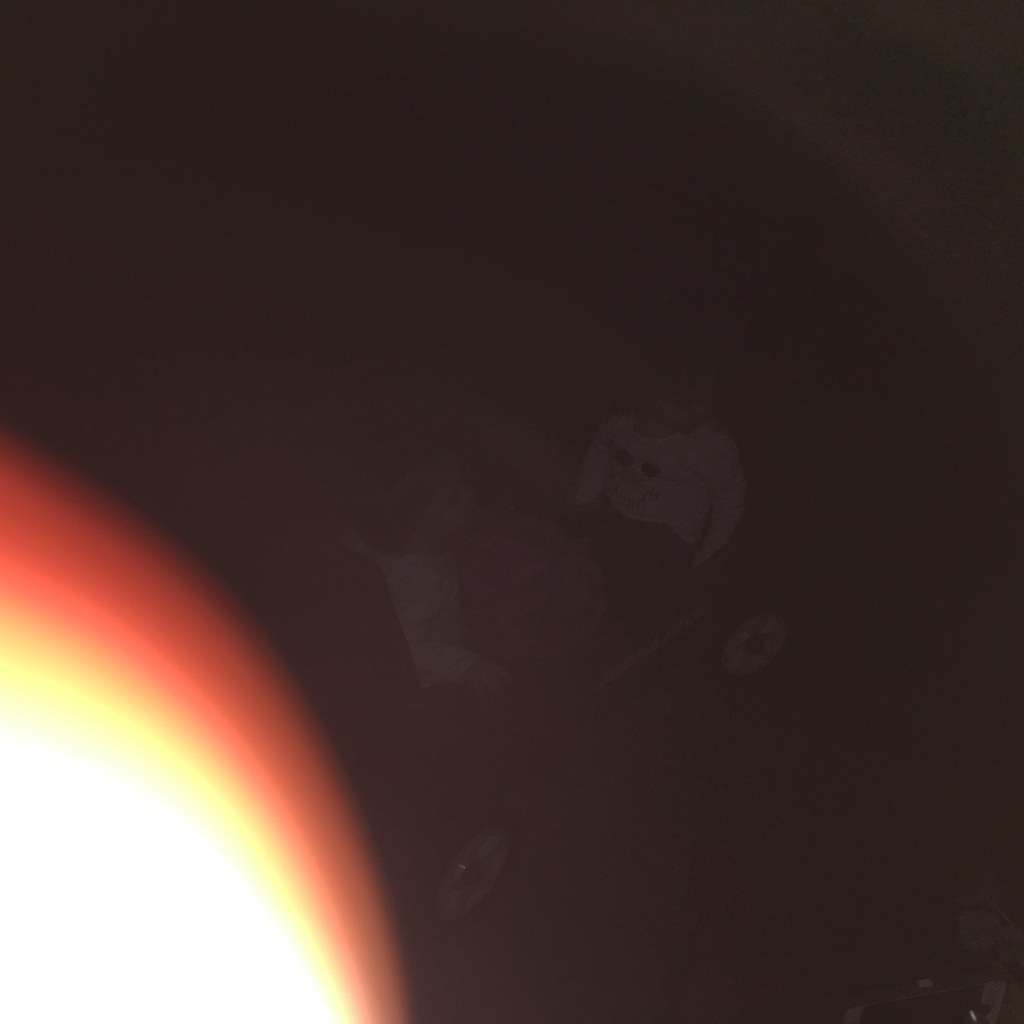In the dimly lit photograph, the majority of the background is enveloped in darkness, but a faint light reveals two children sitting in a vintage red Radio Flyer wagon. The children, who wear white shirts, are positioned facing each other—one on the left side, the other on the right. The wagon's distinctive black wheels with white hubs and a red screw cover in the center can be discerned. A bright, orange-tinted finger partially obscures the bottom left corner of the image, suggesting it was accidentally covering the flash. Amidst the children, a pink backpack is placed, adding a touch of color to the scene. The light from the flash creates halos and bends through the obstruction, casting subtle yellow, orange, and red hues into the shadows.